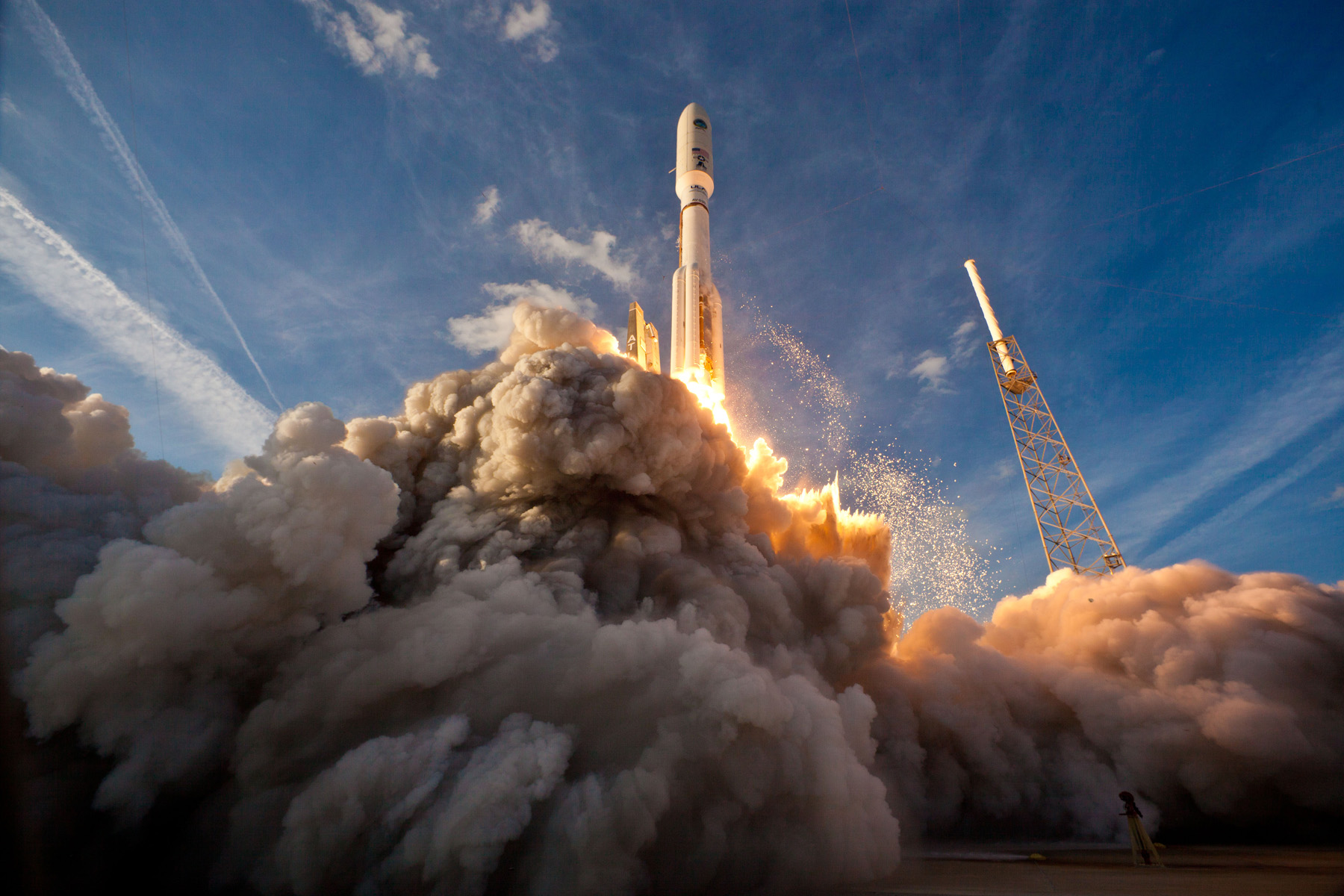The image captures the dramatic moment of a rocket launch, taken from a direct vantage point looking straight up into the beautiful, clear blue sky dotted with a few white wispy clouds. The white rocket, possibly resembling a SpaceX model with its cylindrical body and wider top section, is the central focus as it blasts off vertically. Flames and sparkles burst from its base, cutting through the lower half of the image. Surrounding the lower section of the rocket are immense, billowing clouds of smoke in shades of gray and light brown, spreading across the entire width of the picture. The dense, overlapping plumes create a powerful contrast against the serene sky above. To the right, a red metal tower, likely part of the launch pad scaffolding, stands out. This detailed snapshot captures the intense energy and grandeur of the rocket launch against the calm daylight sky.